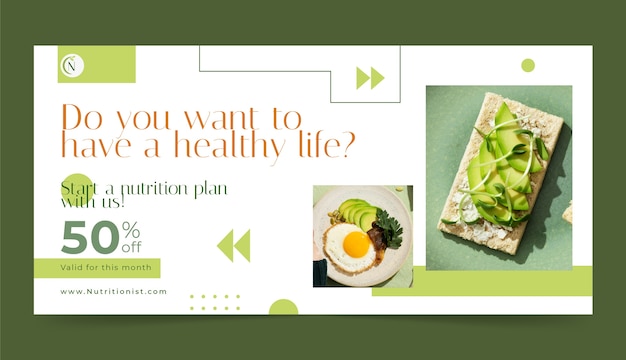The image features an advertisement with a central message asking, "Do you want to have a healthy life?" Encased in an olive green frame, the ad's main area has a white background adorned with various shapes resembling fast-forward and rewind arrows, interspersed with small olive green circles.

Beneath the primary question, the text invites viewers to "Start a nutrition plan with us," followed by a special offer: "50% off, valid for this month." The website, www.nutritionist.com, is provided for further details.

On the right side of the image, there is an appetizing illustration of a nutritious meal. A plate showcases a sunny side up egg accompanied by slices of avocado. Adjacent to this, a flatbread piece is topped with avocado and garnished with sprouts, highlighting a visually appealing and healthy food option.